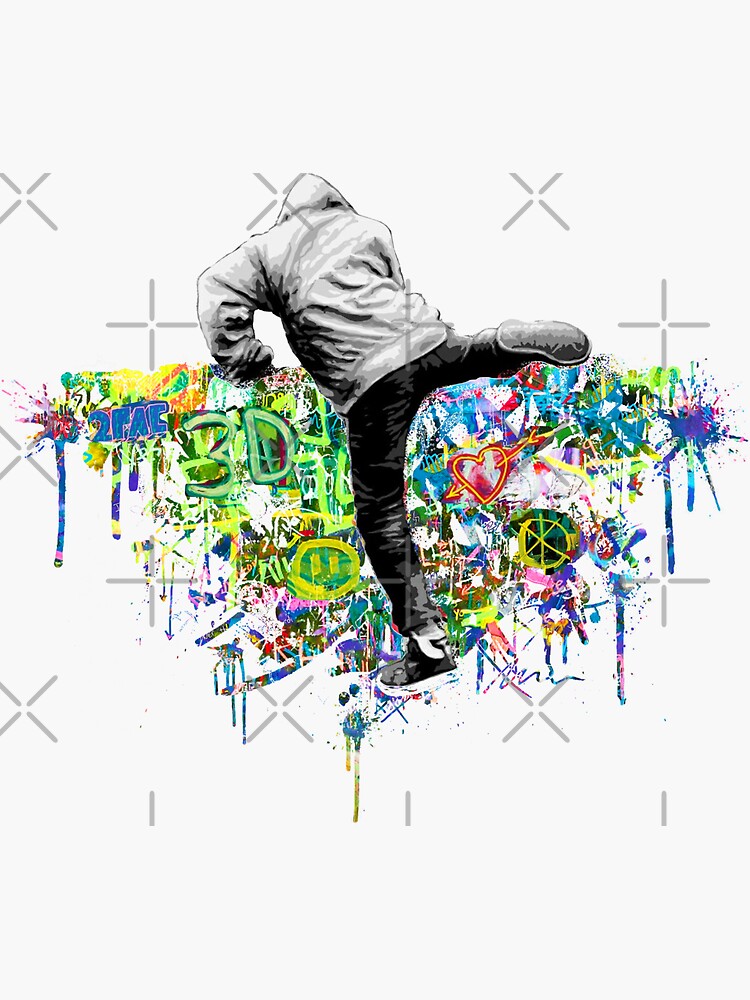The image appears to be either painted or computer-generated with a primarily white background. At the center of this vertically oriented illustration is a man seen from behind, wearing a light-colored hoodie, dark pants, and dark sneakers. He's standing on his left foot while his right leg is extended backward, creating a dynamic pose. His back is to the viewer, obscuring his face, with the focal point on his form.

Behind the man is a vibrant, abstract compilation of graffiti art rich in a variety of colors, such as red, orange, yellow, green, blue, purple, pink, aqua, turquoise, neon green, and neon yellow. This graffiti stretches in an upside-down triangular shape, beginning at the man’s waist and tapering off towards his left foot. The graffiti features a mix of designs, including prominent X marks, smears of blue and green, a 3D "Tupac" in blue, a heart with an arrow, and something resembling a yellow wagon wheel.

Overall, the image melds the monochromatic figure with an explosion of street art colors and shapes, creating a stark and vivid contrast against a white backdrop.